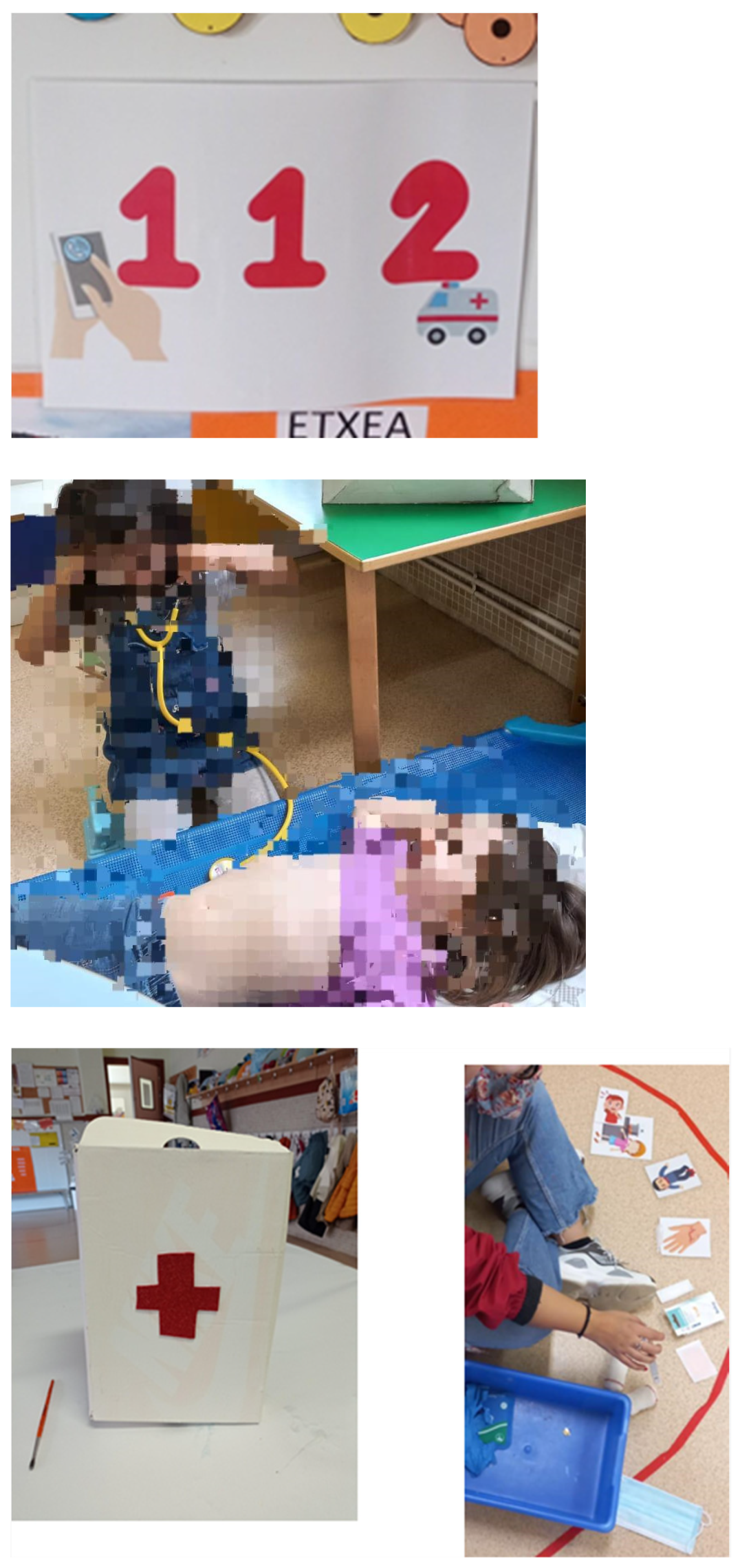The image is a collage of four photographs set against a plain white background, capturing the activities in a kindergarten class. The top photograph is a square close-up of a whiteboard with the number "112" written in magenta and depicts two pale hands tapping on a smartphone, accompanied by an illustration of a white ambulance with a red cross and a red stripe, and the text "E-T-X-E-A" beneath it, suggesting it might be the emergency number equivalent to 9-1-1 in another country. The second photograph shows two pixelated toddlers playing doctor; one is wearing a blue jean outfit and using a yellow stethoscope to listen to the heart of another child in a light lavender-colored shirt who is lying down. The third image, positioned at the bottom left, displays a white medical kit box with a red cross on the front, sitting on a white table. The fourth photograph on the bottom right focuses on a child's feet as they are engaged in playing with cards that have pictures of cats and other items on them, emphasizing playful learning and interaction.